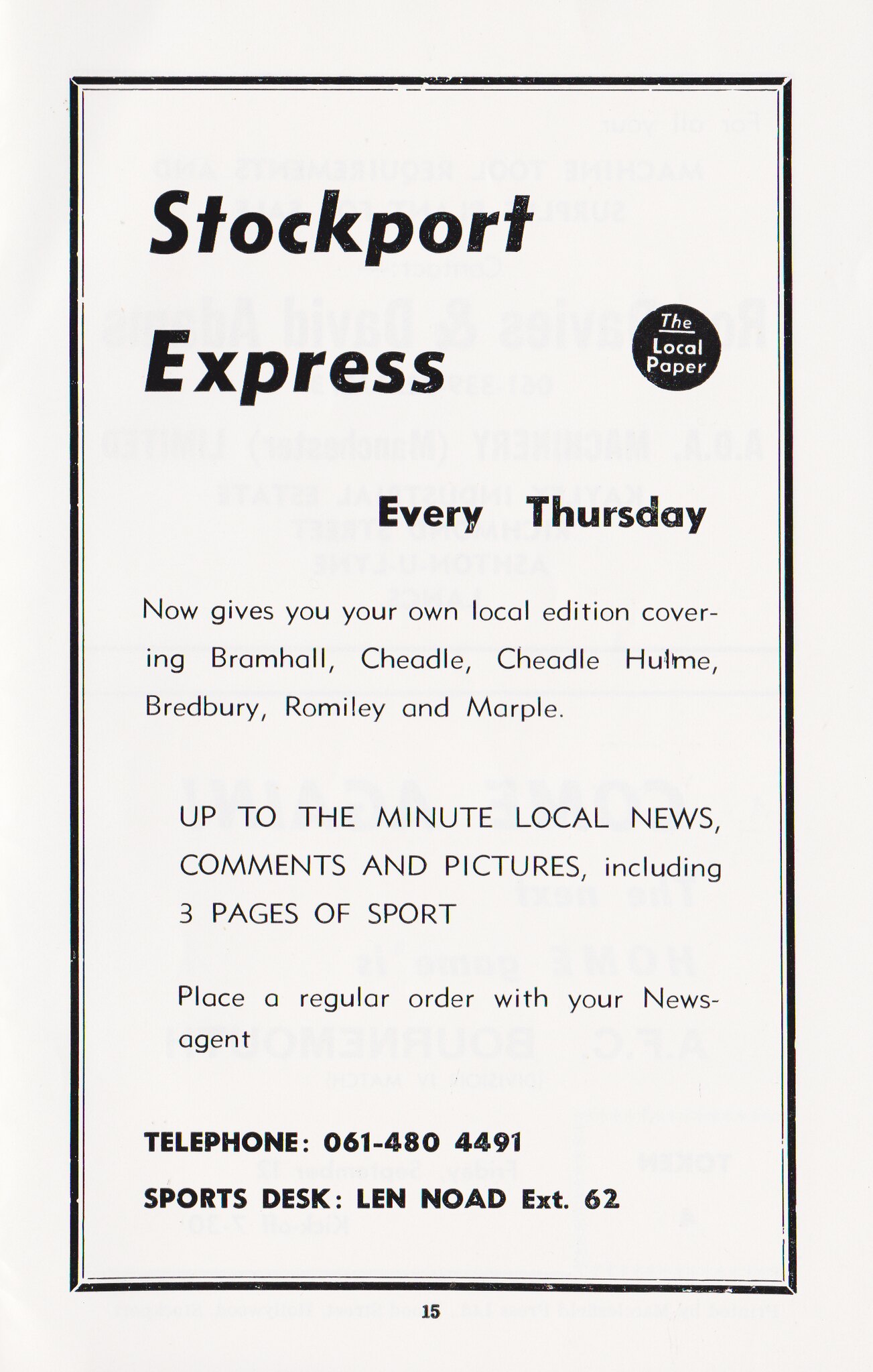The image depicts a vintage advertisement from a slightly yellowed page, numbered 15. At the top, a bold header reads "Stockport Express" against a white background with a black border. Adjacent to this, on the right, is a black circle containing white letters that say "the local paper." Below, in black text, it states "Every Thursday." Further down, small text announces, "Now Gives You Your Own Local Edition, covering Brahell, Chadley, Chadley-Holmey, Bradbury, Raleigh, Miley, and Marple" (with variations in the names indicative of potential printing errors). Prominently, in capitalized letters, the advertisement proclaims, "Up to the Minute Local News, Comments, and Pictures, including three pages of sports." Following this, it advises readers to "Place a Regular Order with Your News Agent." At the bottom, in bold letters, a phone contact is provided: "Telephone 061-480-4491, Sports Desk, Len-Noad, Extension 62." The faded black font and overall design suggest an older publication, possibly from a softcover sports periodical.